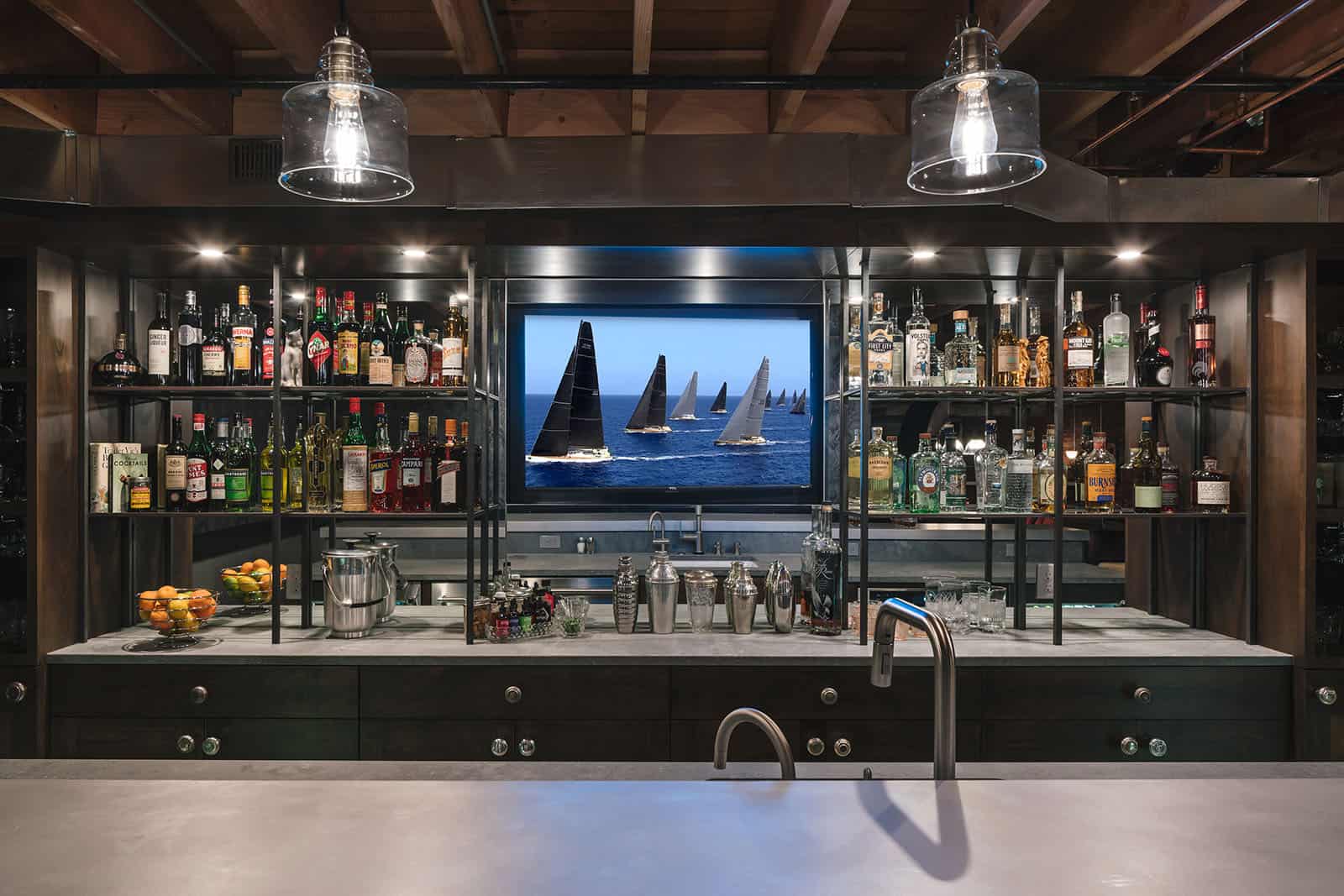In this photograph, we are looking from outside a bar area towards the back wall of what appears to be a private establishment or possibly a bar in a restaurant or club. The foreground features a sleek, white bar counter with two sink faucets curving over a sink behind the bar. Above this, two glass clear lampshades hang from the ceiling, illuminating the scene with a soft light. The rear wall is covered in rich, wooden paneling and adorned with eight shelves divided equally on either side of a central television screen. The television, displaying a sailboat race, is flanked by shelves stocked heavily with high-end liquor bottles. Below these shelves, a countertop runs the length of the wall, holding an assortment of bar tools and accessories, including metal chrome shakers, an ice bucket, a basket of citrus fruits on the left, and empty cocktail glasses on the right. Complementing this setup, the bar area also features black drawers with chrome knobs, adding a touch of modern elegance to the space.